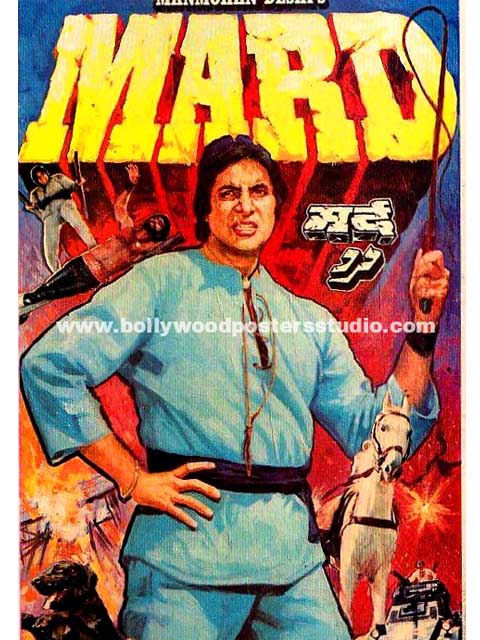The image illustrates an old comic book cover, possibly a movie poster from India, titled "MARD" in bold, yellow block letters with red embossing and black shadows, giving the letters a dynamic, moving effect. Centered across the cover in white font is the URL "www.BollywoodPosterStudio.com." Dominating the scene is an Indian man with short dark hair, garbed in a sky blue tunic and matching pants, secured with a black belt. His facial expression is a grimace, revealing his teeth. He stands in a martial arts-like pose, one hand on his hip and the other wielding a whip with a rope extending from the stick. 

Below his raised elbow, a white stallion charges forward, and behind him, red and orange explosions add intensity to the scene. Near the bottom left, a black dog, possibly a Labrador Retriever, appears with its mouth open and tongue hanging out. On the bottom right, a futuristic tank-like structure with a gun protruding features a person on top, adding an element of high-tech warfare to the illustration. Additionally, another figure lies to the side with black pants and no shirt, reaching upwards as if knocked over. The overall composition is dynamic and action-packed, characteristic of vintage Bollywood dramatic flair.